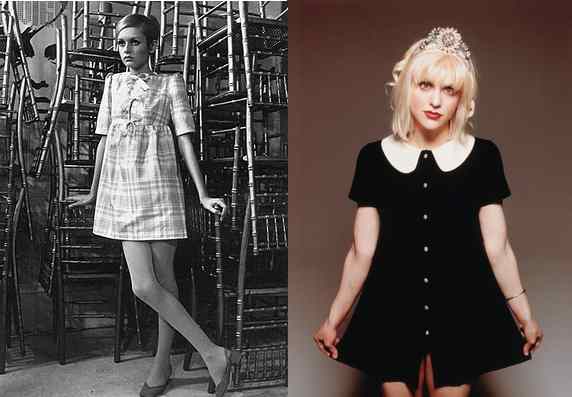The image consists of two photographs placed side-by-side, each showcasing a woman in a babydoll dress. On the left, a black-and-white photograph features a woman with a short pixie haircut and large white earrings, wearing a very short, checkered babydoll dress. She's standing among a pile of stacked bamboo chairs, holding on to the backs of two chairs while her right foot is crossed over her left leg. She has a blank stare, looking off to the left of the frame. On the right, a color photograph of Courtney Love displays her in a black babydoll dress adorned with a white collar and white buttons. Her medium-length blonde hair is messy, complemented by a glossy tiara with a flower design. She has bold red lipstick and is holding out the hem of her dress with both hands against a brownish backdrop.